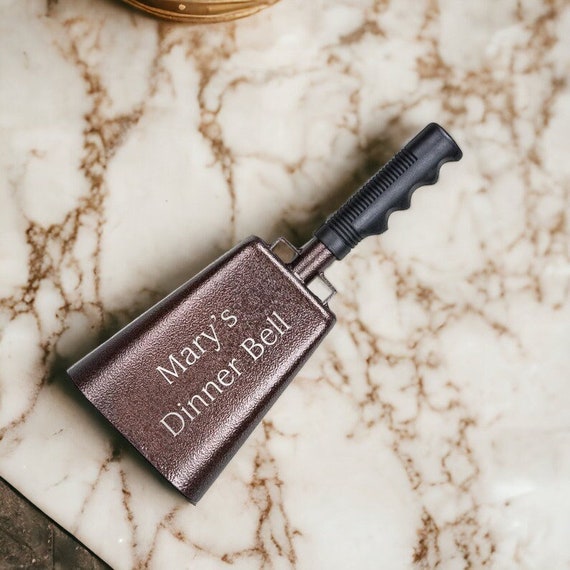This detailed photograph showcases a customized cowbell, prominently labeled "Mary's Dinner Bell" in white text. The bell is crafted from a metallic material, featuring a textured dark gray to black finish with a hint of copper undertones. Its structure is typical of a traditional bell, narrowing at the top and broadening towards the bottom. The bell is equipped with a black rubber handle, designed with finger grips for comfortable holding.

The cowbell is situated on a granite countertop, which has a creamy off-white base with intricate brown veining and inclusions, suggesting both marble and granite characteristics. The surface has a polished, shiny finish, enhancing the overall elegance of the setting. In the photograph, the bell is tilted with the handle pointing towards the upper right corner and the open end of the bell towards the lower left.

Subtle shadowing beneath the bell adds depth to the image, while a small portion of what appears to be wooden table edging is visible in the bottom left corner, hinting that the granite might be part of a cutting board placed on a wooden surface. Additionally, a piece of gold hardware is partially visible at the top edge of the image, adding a touch of curiosity and sophistication to the composition. The overall presentation suggests that this bell, likely used to signal dinner, is both functional and a cherished piece in Mary's kitchen.